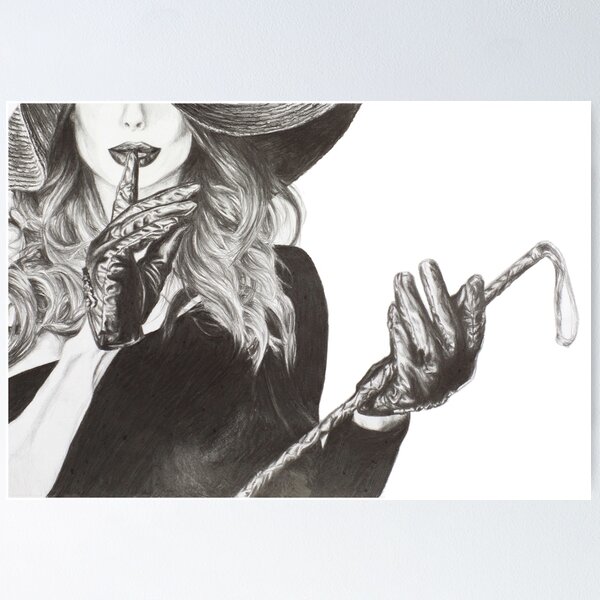This black-and-white drawing features a woman depicted from the waist up to just below her eyes, which are not visible due to the cropping of the image. She appears to be a white woman with long, curly shoulder-length hair and a narrow nose, wearing a large hat, possibly straw or resembling a babushka style. She dons a distinctive black dress, which covers her left arm entirely while leaving the right arm sleeveless. Both hands are gloved in black leather, contributing to a seductive aura. Her right hand is poised with her index finger pressed to her lips in a "shhh" gesture, while her left hand holds what looks like a whip or a stick with a string attached. The background remains a blank white expanse, accentuating her figure which is positioned slightly left of center. This rectangular drawing is framed by lighter gray edges, enhancing the central white background where the woman captivates focus.